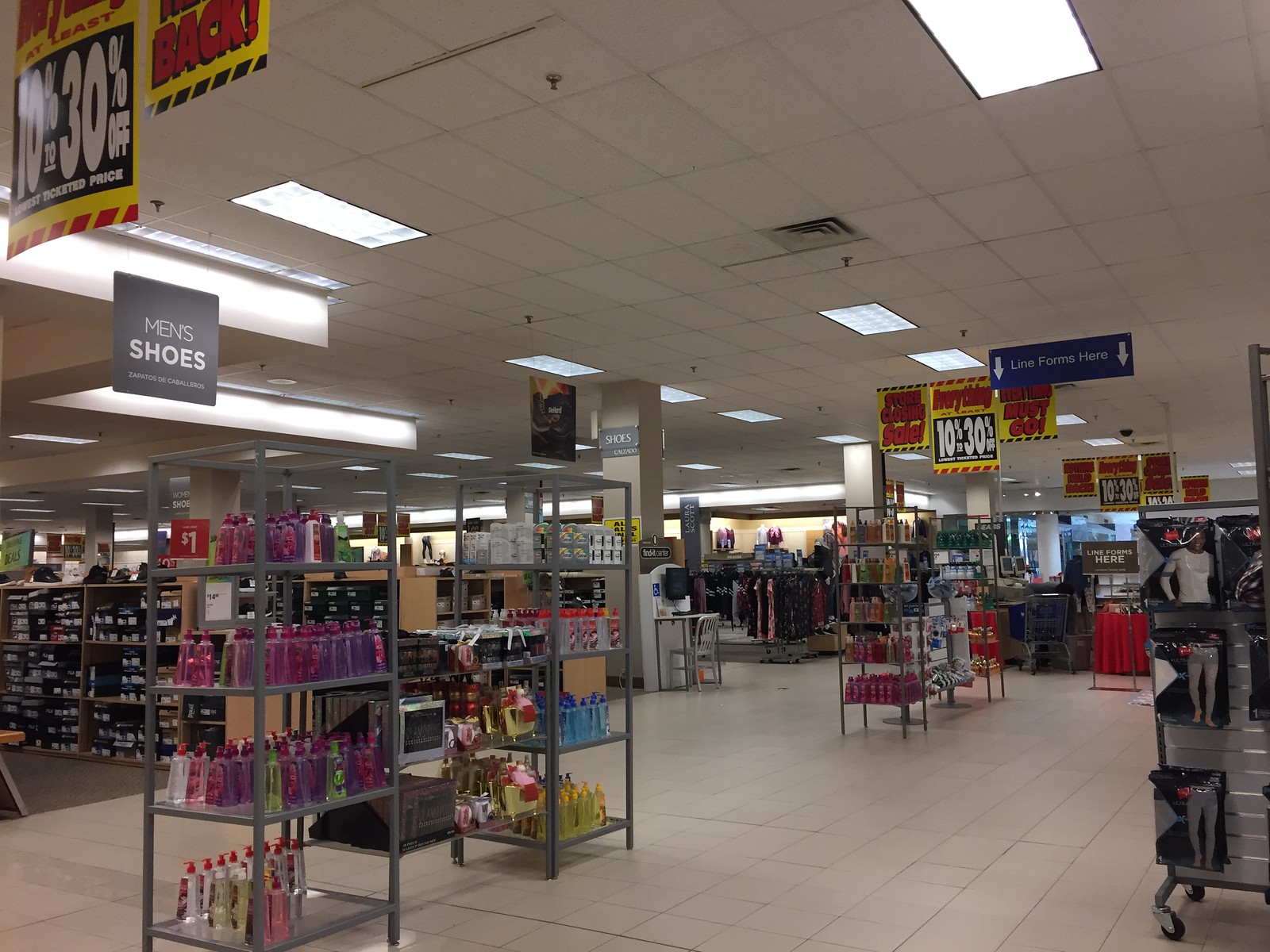The image depicts the interior of a sprawling big-box variety store adorned with signs of an ongoing sale, suggesting discounts ranging from 10% to 30%, possibly indicating a clearance or going-out-of-business event. Various shelves stocked with items such as shampoos, lotions, men's shoes, and tights can be seen. The upper left corner features hanging banners announcing the sale. In the background, racks of clothing stretch into the distance, indicating a wide assortment of apparel. On the right side, there are displays of long johns and long-sleeved insulated tops. Higher-end items, such as clothing on mannequins, are showcased in illuminated cabinets towards the back. The store has a tile floor and recessed lighting set into an acoustical tile ceiling, which shows signs of age with visible stains around the vents. Overall, the image captures the eclectic range of merchandise typical of a variety store facing significant markdowns.